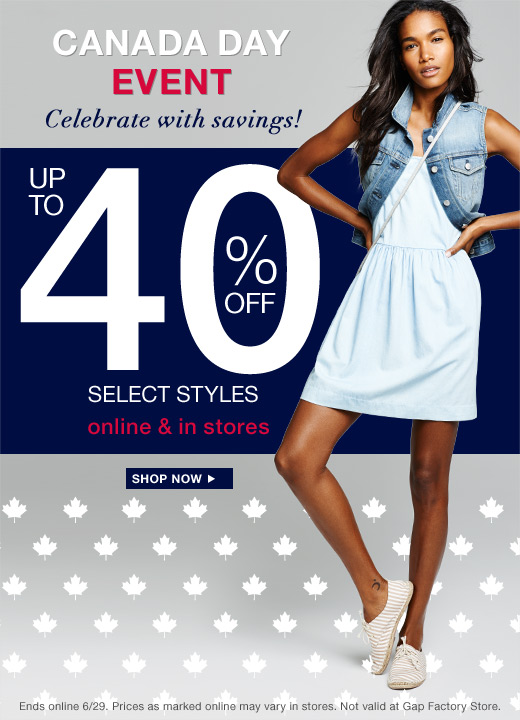The image showcases an advertisement set against a grey background. In the top left corner, the words "Canada Day" are prominently displayed in white lettering. Below this, the word "EVENT" stands out in bold red letters. Following this, the phrase "CELEBRATE with savings!" is written in navy blue font. 

On the right side of the advertisement, there is a young woman with brown skin and black hair. She is dressed in a stylish ensemble, featuring a white dress paired with a blue jean jacket vest that includes pockets at the top and buttons down the front. She has a bag slung across her shoulder, with only the strap visible. The woman strikes a casual pose, with one leg straight and the other bent, her foot resting against her straight leg.

Centrally placed within a navy blue rectangle, bold white text announces "Up to 40% off," with "SELECT STYLES" written in smaller white font just below. Further down, the text "ONLINE AND IN STORES" is also in white. At the bottom, a grey rectangle featuring a small Canadian maple leaf contains a call to action with the words "SHOP NOW" prominently displayed.